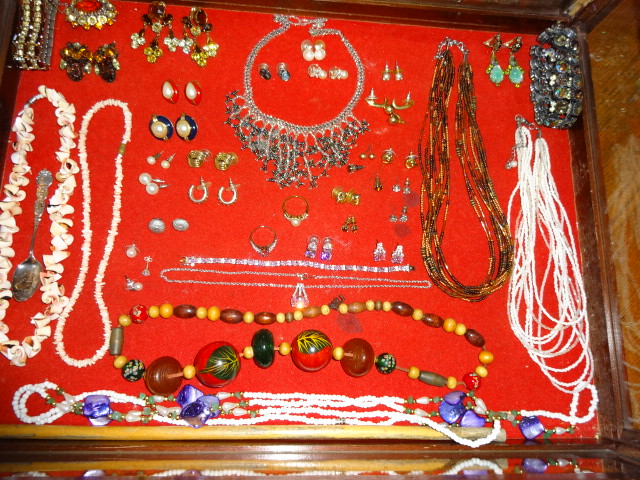The image presents a detailed, overhead view of a large, square jewelry case framed in wood with a vivid red felt interior. The case houses an extensive and assorted collection of jewelry, meticulously arranged but without a specific theme. At the bottom, a white beaded necklace stands out, layered beneath another beaded necklace adorned with various red, yellow, and mauve trinkets. Above these, there is a delicate necklace made of white stones. Flanking these central pieces are an assortment of different beaded objects, including what appears to be a shell necklace with a spoon nestled within it. Adding to the variety, there are numerous earrings, including stud and pearl varieties, distributed throughout the display. The arrangement also features several distinctive items like brooches, costume jewelry, rings with pearl and amethyst-like stones, and a unique necklace from which multiple bangles dangle. The jewelry, seemingly pinned to the case, conveys an eclectic mix often seen in flea markets, museums, or personal collections, each piece contributing to the diverse and vibrant display.